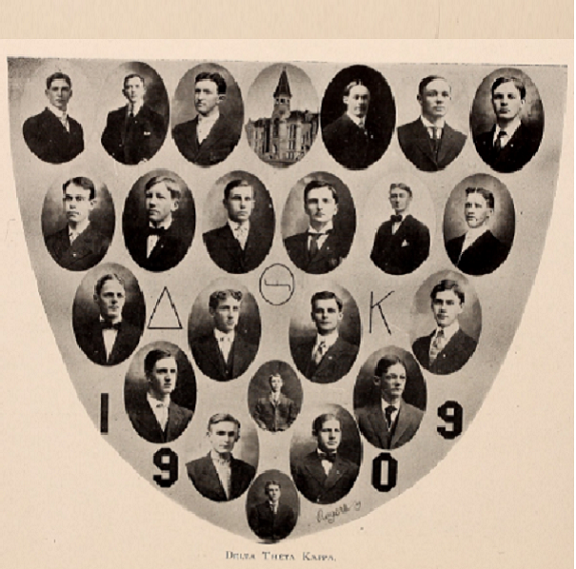This is a sepia-toned, vintage image from what seems to be a yearbook, showcasing a fraternity group from 1909. The central design of the image is a shield-like shape, filled with around 20 to 25 oval portraits of young men, all dressed in black suits with white shirts and either ties or bows. In the top row center, a notable oval image features a building with a steeple. Surrounding these portraits are various Greek symbols; notably, a combination of a triangle, an 'O', and a 'K' appears centrally among the images. At the base of the shield, curving along its edge, the year '1909' is inscribed. The year is split with '19' on the left and '09' on the right. Below this, it reads "I Beta, Theta, Kappa," indicating the fraternity's name. The entire shield motif stands against a light tan or beige rectangular background, giving it an antique and distinguished appearance.